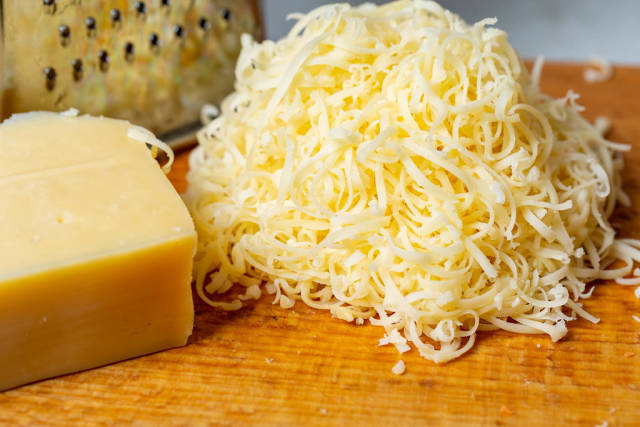The image is an indoor, close-up shot of a block of Parmesan or similar hard cheese positioned on a chopping board with a small, slightly rusty cheese grater in the background. The cheese on the left is off-yellow and appears darker on the sides, indicating its hard texture. Adjacent to the block is a mound of finely grated cheese resembling thin, hair-like strands. The chopping board displays a crosshatched pattern, lending a rustic feel to the composition. The background, including a subtle blue wall, is intentionally out of focus, drawing attention to the central objects—the cheese block and the grated cheese pile. The excellent lighting emphasizes the textures and colors, making the cheese the focal point of the image.